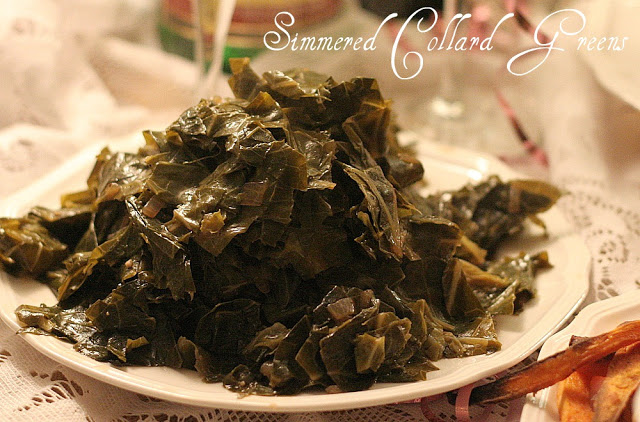In this detailed image, a large circular white porcelain plate is prominently positioned near the center, slightly towards the bottom. The plate is heaped with dark green collard greens, described as almost resembling a mountain of vegetables, showcasing their freshness and readiness to eat. The plate is set on a white, possibly lace, tablecloth, suggesting a table setting which could be in a kitchen or a restaurant. In the top right corner of the image, fancy white text reads "Simmered Collard Greens," indicating the dish. Additionally, in the bottom right corner of the image, a few orange sweet potato fries are visible, adding a pop of color. The overall color palette includes white, brown, orange, yellow, green, and pink, creating a vibrant and appealing visual. A pitcher or glass with a green bottom is also faintly visible in the background, hinting at a casual dining or menu presentation setting.